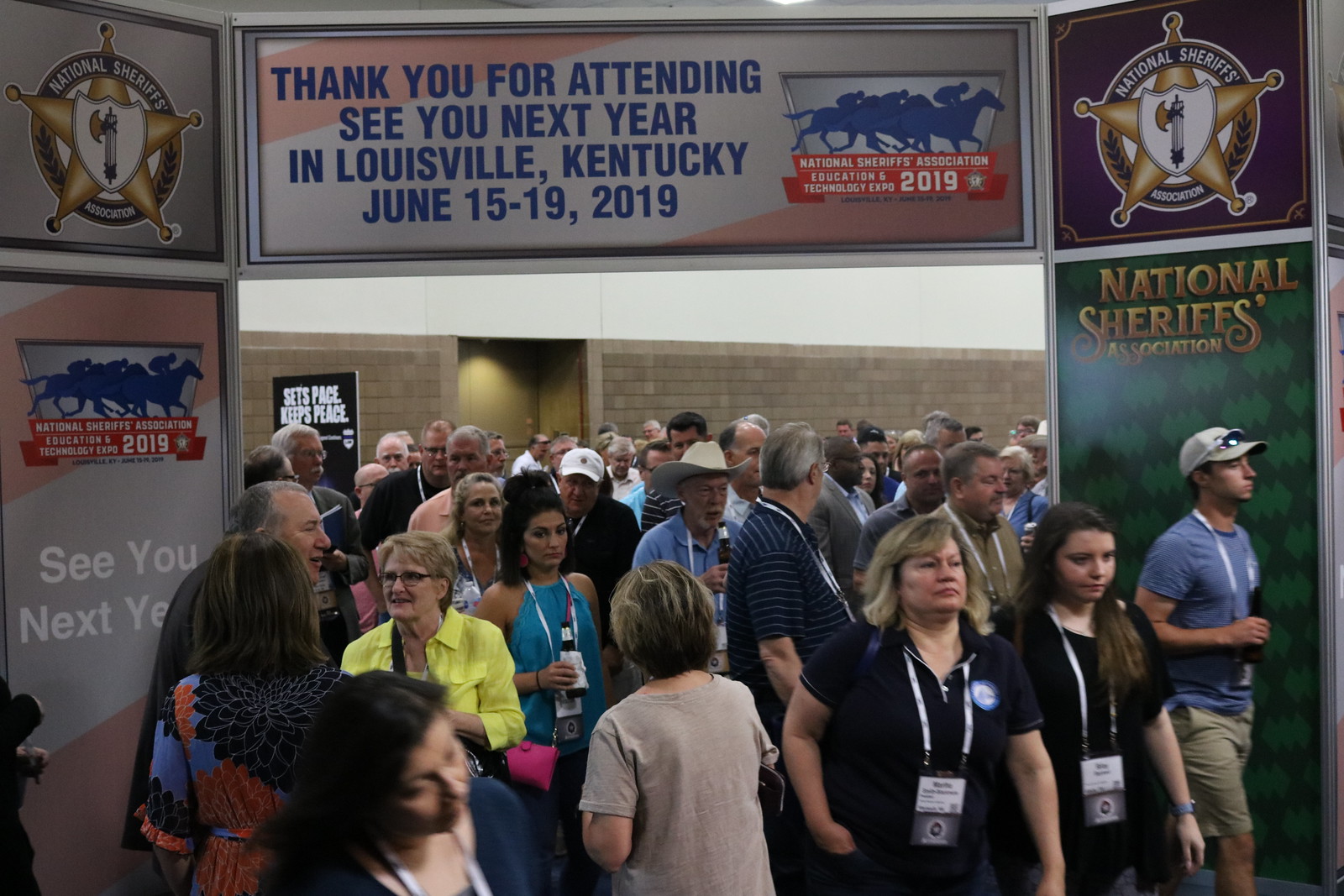The image depicts a large, diverse crowd of 40 to 50 attendees exiting the National Sheriff's Association Education and Technology Expo 2019. The scene is set against a backdrop of a brick wall with a door, within an alcove that features an artificial arch, possibly erected for the event. Prominently displayed above the crowd are banners that read, "Thank you for attending. See you next year in Louisville, Kentucky, June 15 to 19, 2019," and the event name along with the organization's logo. The attendees, comprising various races, ages, and genders, are identifiable by neck lanyards and tags typically worn at conventions. Notably, one individual in the center of the crowd is wearing a cowboy hat, highlighting the variety in attire. The overall atmosphere is bustling, typical of a convention as people move in and out of the building through large doors.